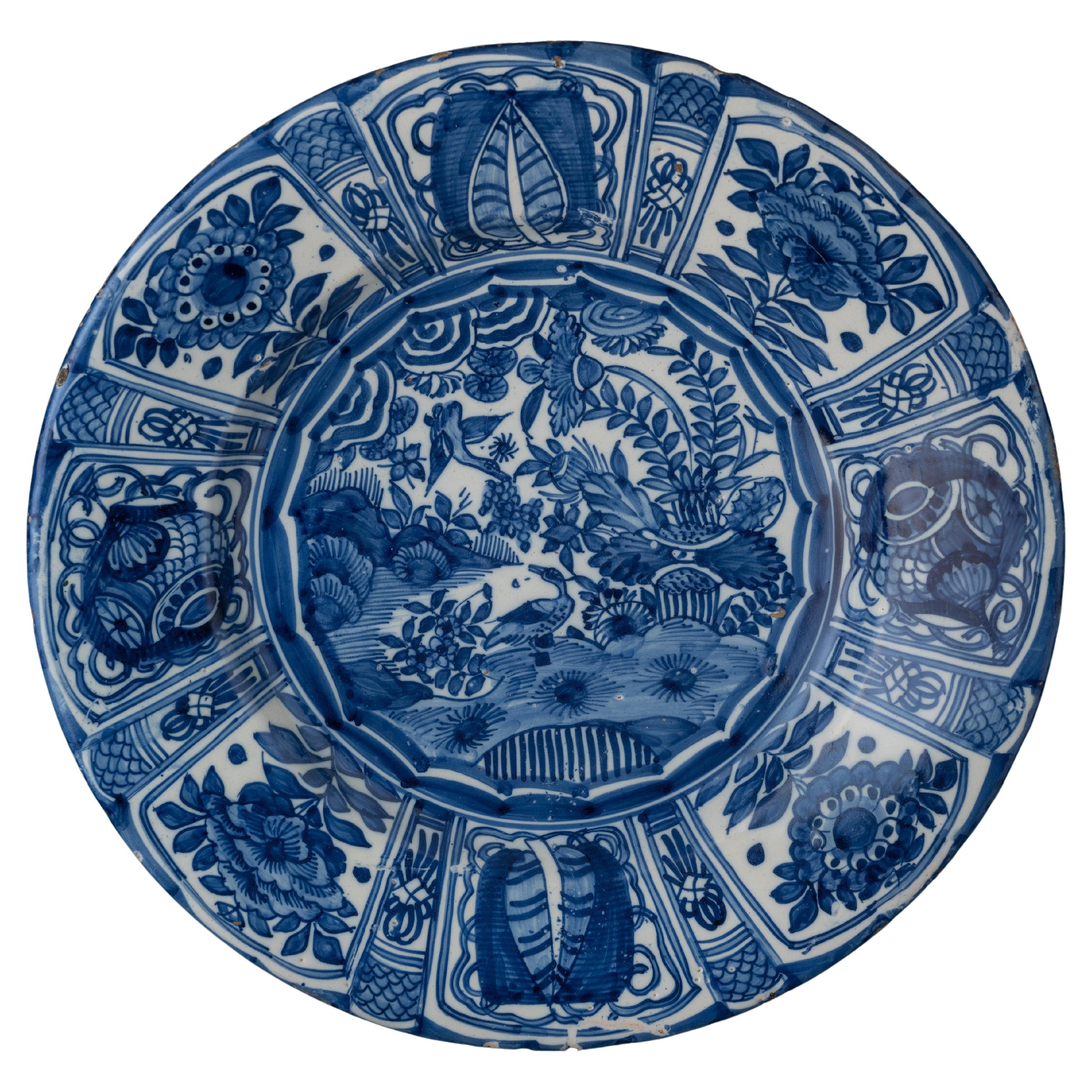This is a well-focused, close-up photograph of an antique decorative plate, set against a white backdrop. The plate is predominantly blue on a white background, featuring intricate and delicate designs. The central portion of the plate depicts a serene outdoor scene: a duck standing on a shore surrounded by various plants, flowers, and possibly a couple of birds, rendered in darker shades of blue with hints of lighter blue. Surrounding the central image, the edge of the plate alternates between larger, detailed images of different types of flowers and leaves, separated by smaller decorative designs and squiggly lines. The overall design has an aquatic and natural theme, with additional symbols like leaves, berries, and circles adorning the plate. Notably, the plate has a small hole at the top, indicating it was likely hung as a decorative piece. Despite a few chips and minor damage at the bottom, the antique china plate appears to be well-preserved.